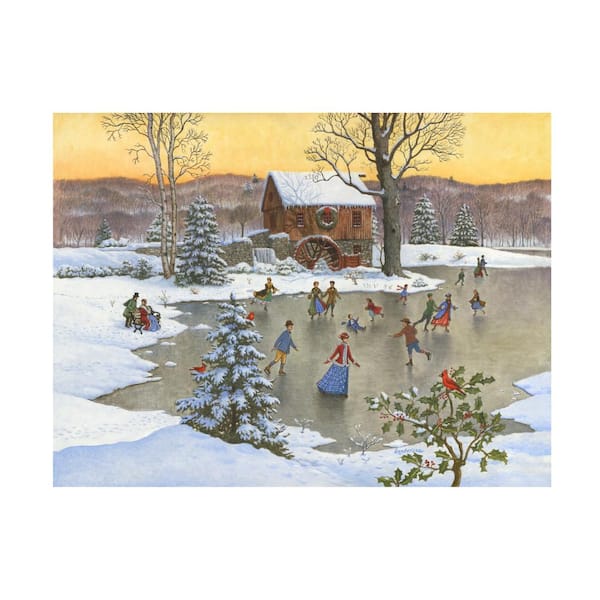This richly detailed rectangular painting captures a lively winter scene set during sunset, evident from the orange-yellow hues illuminating the sky. Dominating the center is a frozen pond, bustling with roughly a dozen ice skaters dressed in colorful attire. Notable figures include a woman in a blue skirt, white shirt, and red coat, a person in yellow pants and a blue coat, and a couple holding hands as they skate. One skater is depicted falling, with another hurrying to assist. A child with a flying scarf skates in the background, adding to the dynamic activity on the ice.

Encircling the pond are snow-covered banks and two lush evergreen trees on the left, each adorned with cardinals. The snowy foreground on the right side features a holly tree with red berries, on which another cardinal perches. Here, a snow-dusted evergreen stands adjacent.

In the background, a quaint brown house with a pitched, snow-covered roof and a waterwheel, suggesting a mill, overlooks the scene. A wreath with a red ribbon decorates its wooden upper part. Flanking the house, two larger trees stand bare, framing the idyllic winter tableau. Beyond the house, brown rolling hills and leafless trees form a silhouette against the vibrant sky, completing the serene yet bustling winter setting. A bench on the left hosts a seated woman observing the skaters, while a man stands behind her with hands resting on the bench. A small waterfall flows near the base of the mill, adding a touch of natural charm to the idyllic winter landscape.